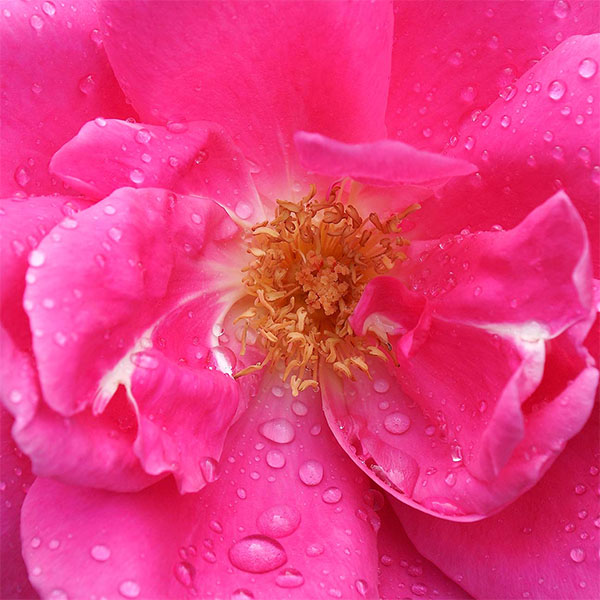The image is a high-quality close-up of a vibrant pink flower, likely a rose or a peony, with its petals spread out across the entire frame, leaving the edges of the flower and stem out of view. The composition centers on the flower's core, where a cluster of slightly dried golden stamen is fully visible. The petals, predominantly fuchsia pink with subtle white striations on the inner ones, dominate the scene, making up 90% of the photo. Each petal is adorned with water droplets, giving the appearance of being dew-kissed or just rained on, with one petal even showing a small pool of water. The image captures the fresh, natural beauty of the flower without any text or people present, focusing intently on the detailed and delicate textures of the petals and stamen.